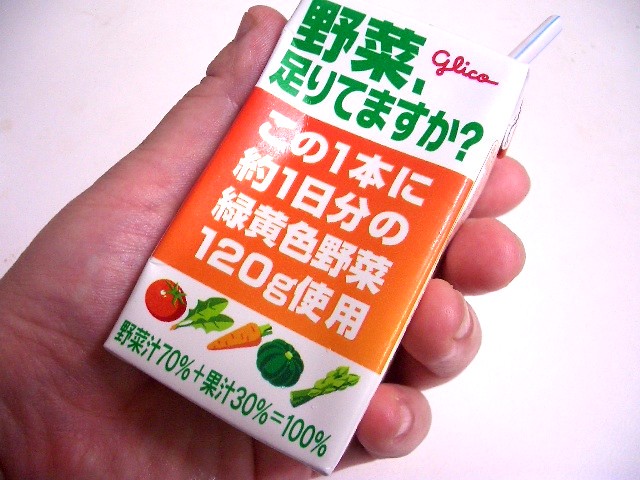In a close-up, cleanly manicured left hand, a man holds a well-used juice box adorned with Japanese characters against a plain white background. The juice box features a red cursive "Glico" at the top, signaling the brand. It has a white body with an orange rectangle in the middle, below which colorful illustrations of various vegetables like a tomato, leafy green vegetable, carrot, squash, and asparagus are displayed. A white straw with blue stripes sticks out from the top, indicating it has already been used. The box label reads "70% + 30% = 100%" in bold numbers alongside the vibrant illustrations. The bottom of the orange rectangle prominently displays "120 grams" in white letters.